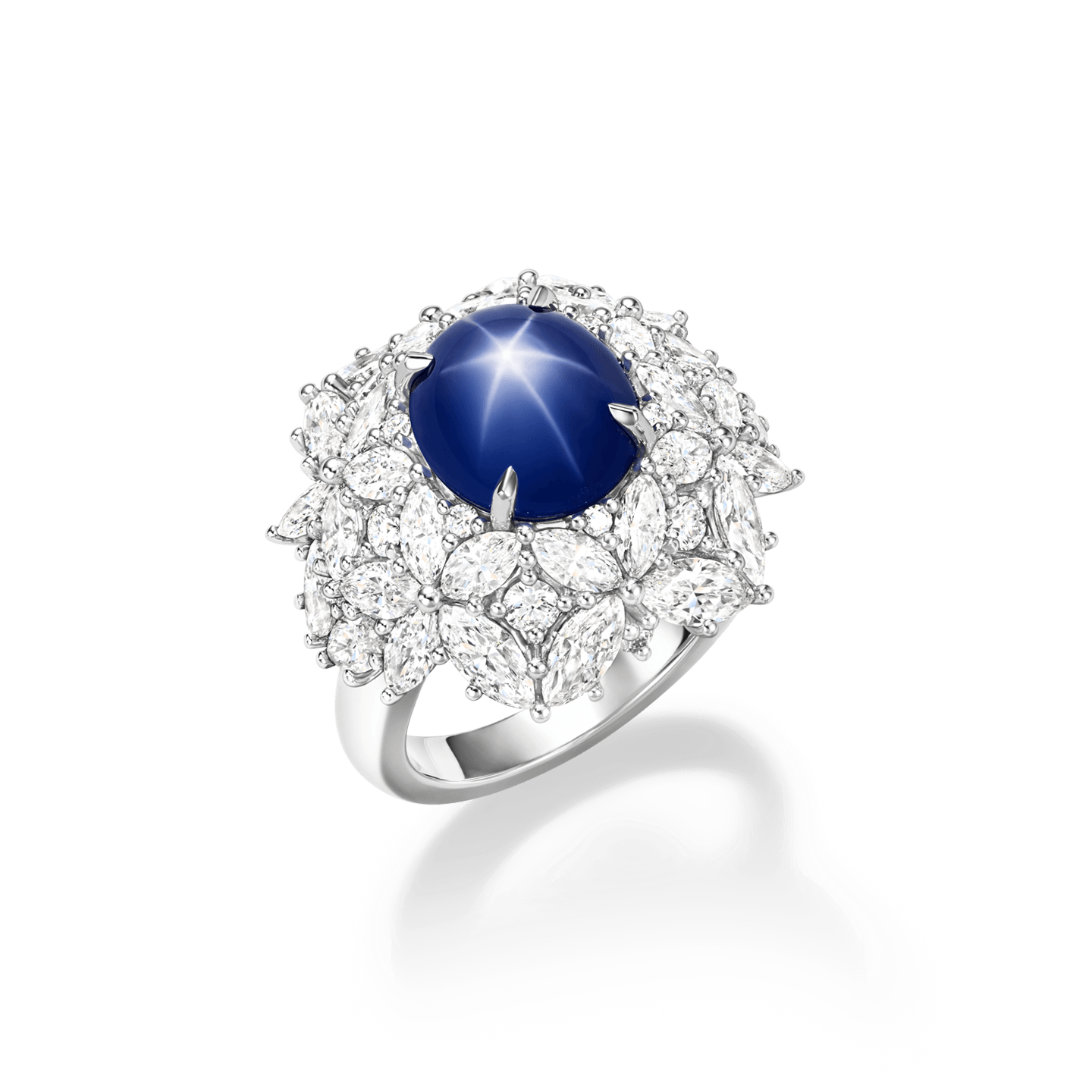This is a detailed close-up photograph of a silver-toned diamond ring featuring a stunning arrangement that's both intricate and elegant. At the center of the ring is a striking dark blue gemstone, which is surrounded by numerous white diamonds, possibly creating a floral-like pattern. The blue stone is intricately held in place by four clasps, positioned in pairs at 90-degree angles. The blue gem itself features a white starburst pattern, with a small circle at the center and six lines emanating from it, reminiscent of something you might see in the night sky. The ring is positioned upright on a white surface, and it appears to be either glued or digitally depicted with careful attention to detail. A light source from above casts a subtle reflection on the blue gemstone, accentuating its three-dimensional quality and adding depth to the image.